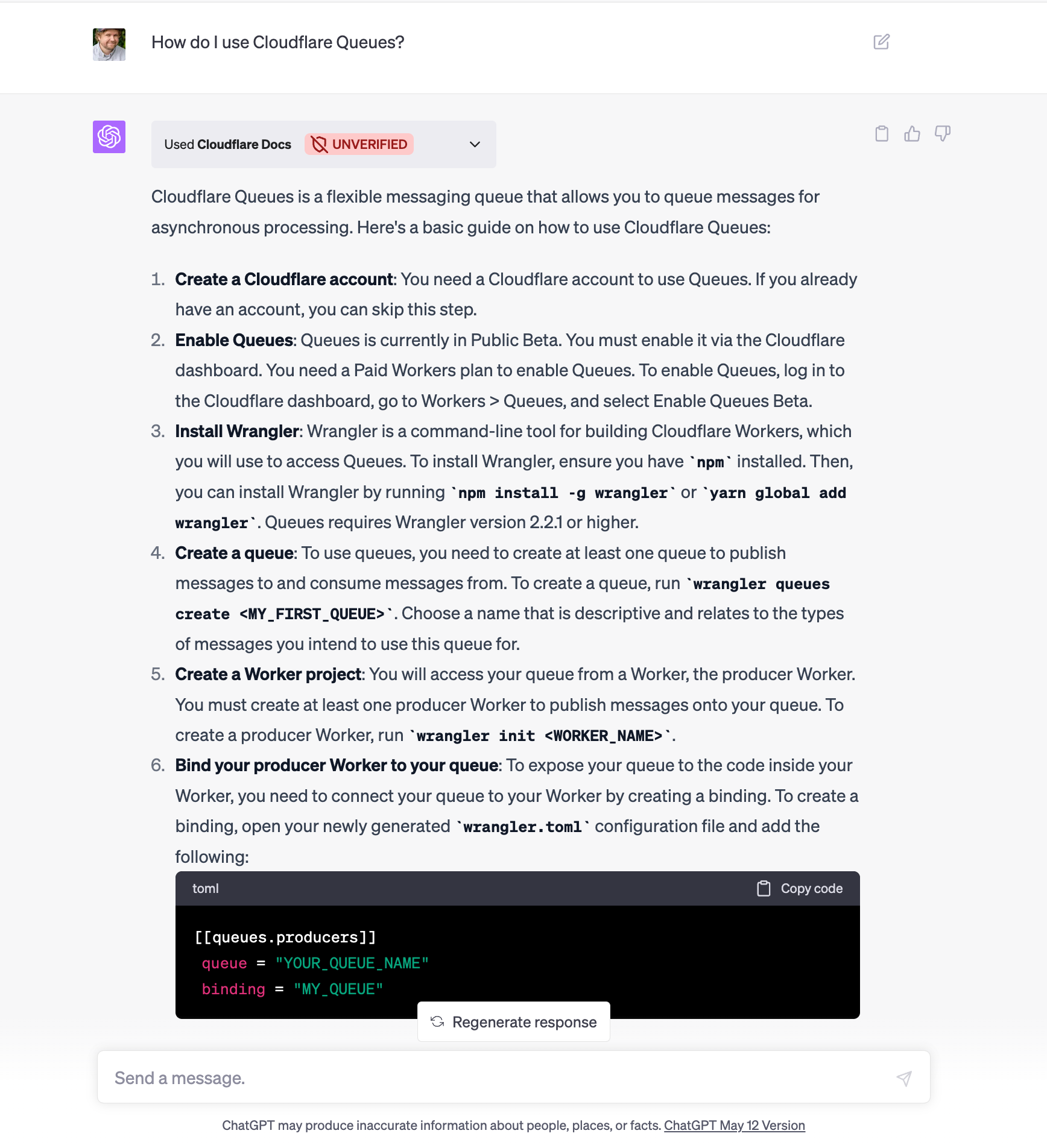A detailed caption for the provided image could be:

---

This image is a screenshot of an interactive Q&A webpage hosted by ChatGPT, specifically from the May 12 version. At the very top of the page, there's a prominent search box alongside a small profile picture icon. Below, in a central panel, a user has queried, "How do I use Cloudflare queues?"

Accompanying the user's query is a response from the ChatGPT system. Next to the query, a small but distinct purple icon with intricate white designs is present, labeled "use Cloudflare docs." Directly beneath this icon, within a red and light red notification box, the word "unverified" is prominently displayed.

The response provided by ChatGPT begins with an explanation: "Cloudflare Queues is a flexible managing queue that allows you to queue messages for asynchronous processing. Here's a basic guide on how to use the Cloudflare queues." This introduction is followed by six detailed step-by-step instructions, each written in black text.

Located in the top right corner of this answer section are interactive thumbs up and thumbs down icons for user feedback, along with a trash can icon that seemingly allows users to delete the response. 

Additionally, towards the bottom right of the image, there's a black box with prominently highlighted green and red text, offering the option to "regenerate response."

Lastly, at the very bottom of the screenshot is a small disclaimer stating, "ChatGPT may produce inaccurate information about people, places, or facts."